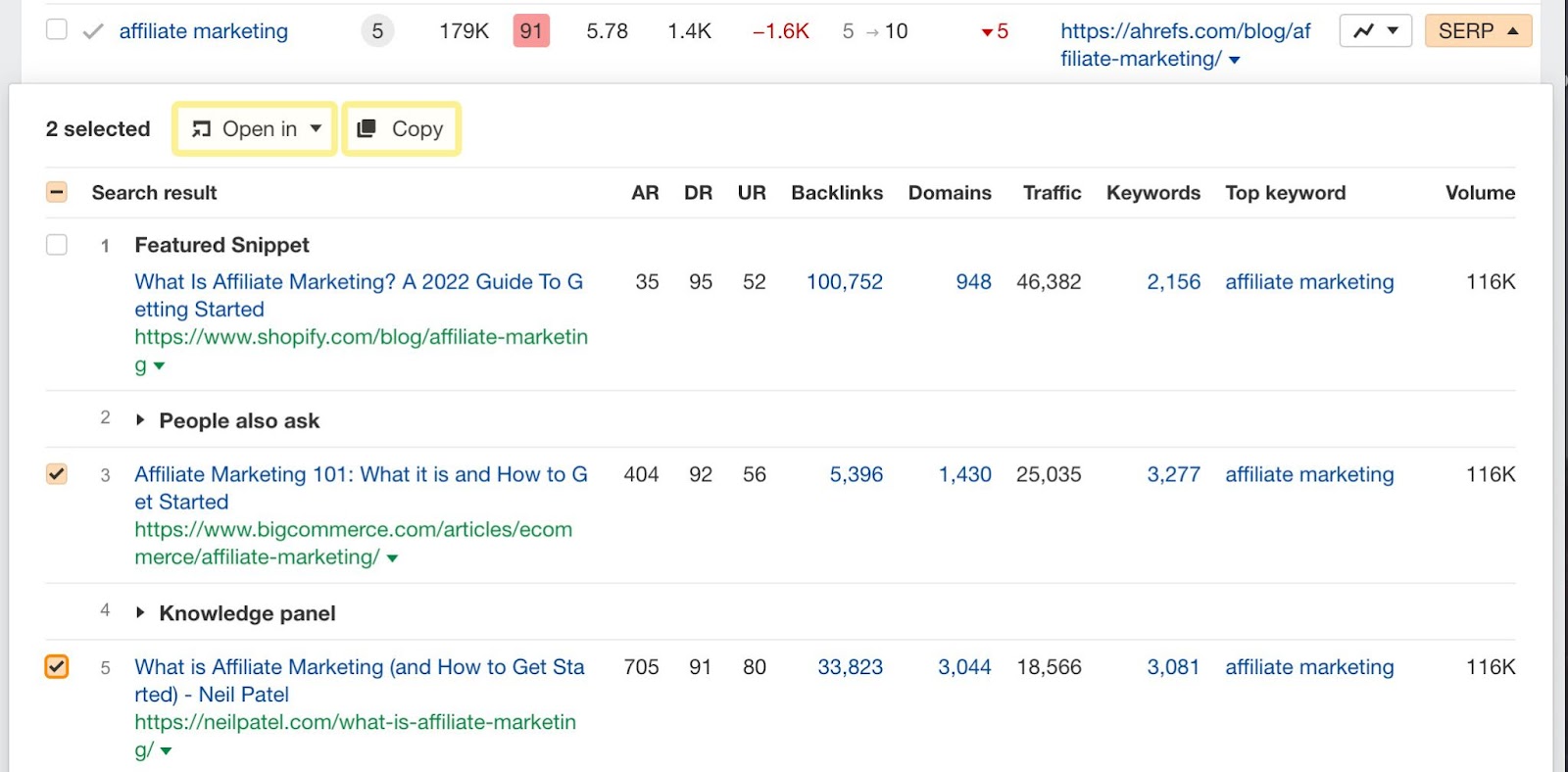**Detailed Caption:**

The image features a detailed user interface with various elements framed by a border on the left and right sides. In the top left corner, there is a small square icon followed by a check mark, and adjacent to it, the text "Affiliate Marketing" appears in blue. Below this, there are multiple data points: a shaded circle containing the number 5, the figure 179,000, a pink block displaying 91, and the sequence 5.78, 1.4K, -1.6K, 5, - 10. A red downward arrow followed by the number 5 is also present. 

Next, there is a URL: "ahrefs.com/blog/affiliate-marketing/". On the following line, the URL continues with "filtrate-marketing/" and is followed by another downward arrow. 

At the bottom right, there is an orange-colored box with the acronym "SARP" in uppercase letters, accompanied by an upward arrow. To the side, there are two selection options within yellow-bordered boxes: one labeled "Open in" and the other "Copy."

Prominently displayed are result categories such as one "Featured Snippet," "People Also Ask" questions, and the title "Affiliate Marketing 101: What it is and How to Get Started," with the word "Started" moving onto a second line. Lastly, a "Knowledge Panel" section is identified. All text within these sections appears in black.